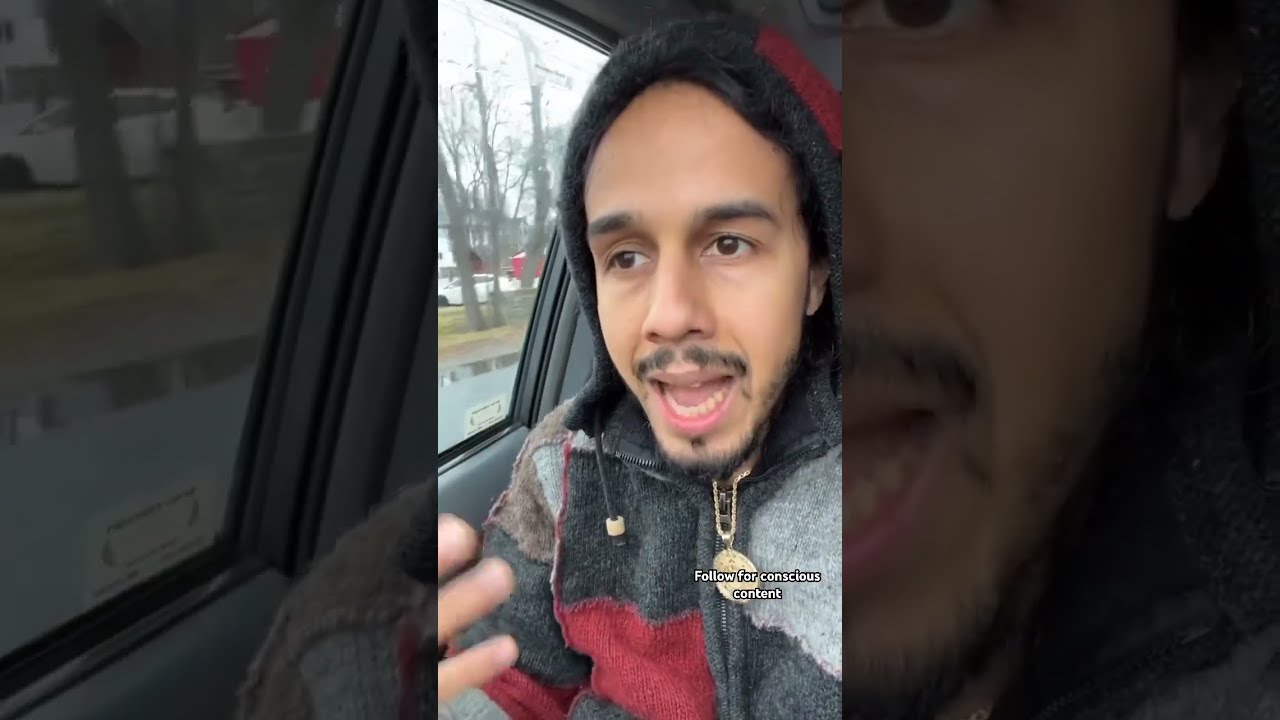A detailed photograph captures a man seated in the passenger side of a car, gesturing with his right hand and speaking, as his mouth is slightly open revealing his bottom teeth. He has a dark complexion, brown eyes, and wears a beard and mustache. His head is covered with the hood of a fleece hoodie, which is a mix of dark gray, light gray, and red squares. The hoodie has a gold zipper with a circular gold attachment, and he also dons a gold necklace with a noticeable pendant. The image is framed by two enlarged, grayed-out panels on the sides, which magnify elements of the central picture. Through the car window, one can observe tall, barren trees and a white car passing by under a dull gray sky, suggesting a winter setting. There is a faint text near the zipper that seemingly reads “follow for conscious content.”